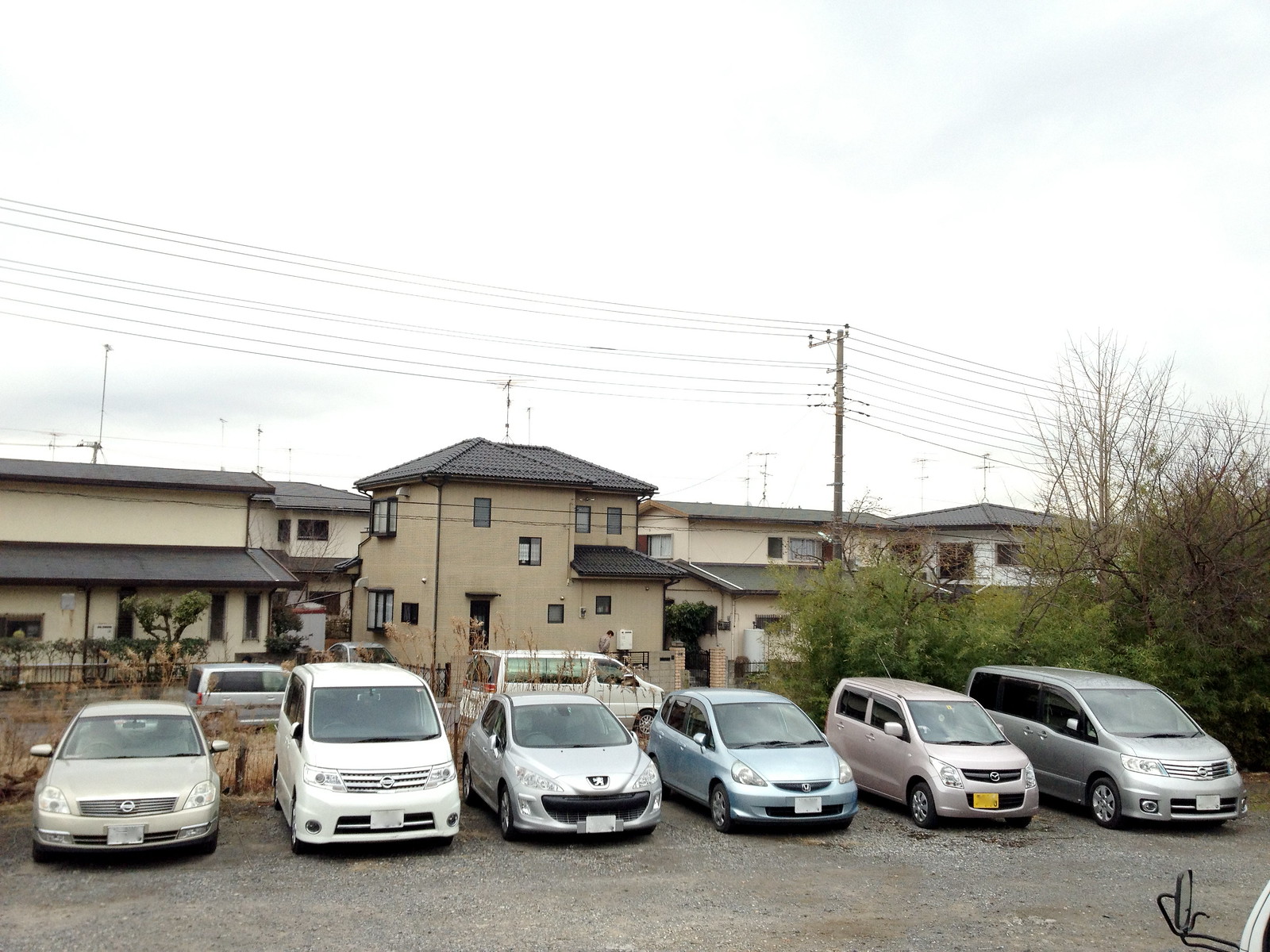In this photo, a group of six vehicles is parked in a gravel-covered parking lot in front of a series of tan-colored buildings with brown rooftops. The vehicles, comprising mostly of vans and sedans, are lined up facing the viewer. From left to right, there is a sedan, a van, a smaller sedan, a light blue hatchback, a box-style car, and a minivan. The cars are of various colors: primarily shades of white and gray, with a standout blue vehicle and a champagne gold-colored van. The two vehicles on the right are seen from a diagonal front and side perspective. The parking lot features some black lines toward the bottom right corner, and there are a few bushes and trees located to the right. Power lines and their poles are visible in the background against an overcast sky, with a hint of blue peeking through.